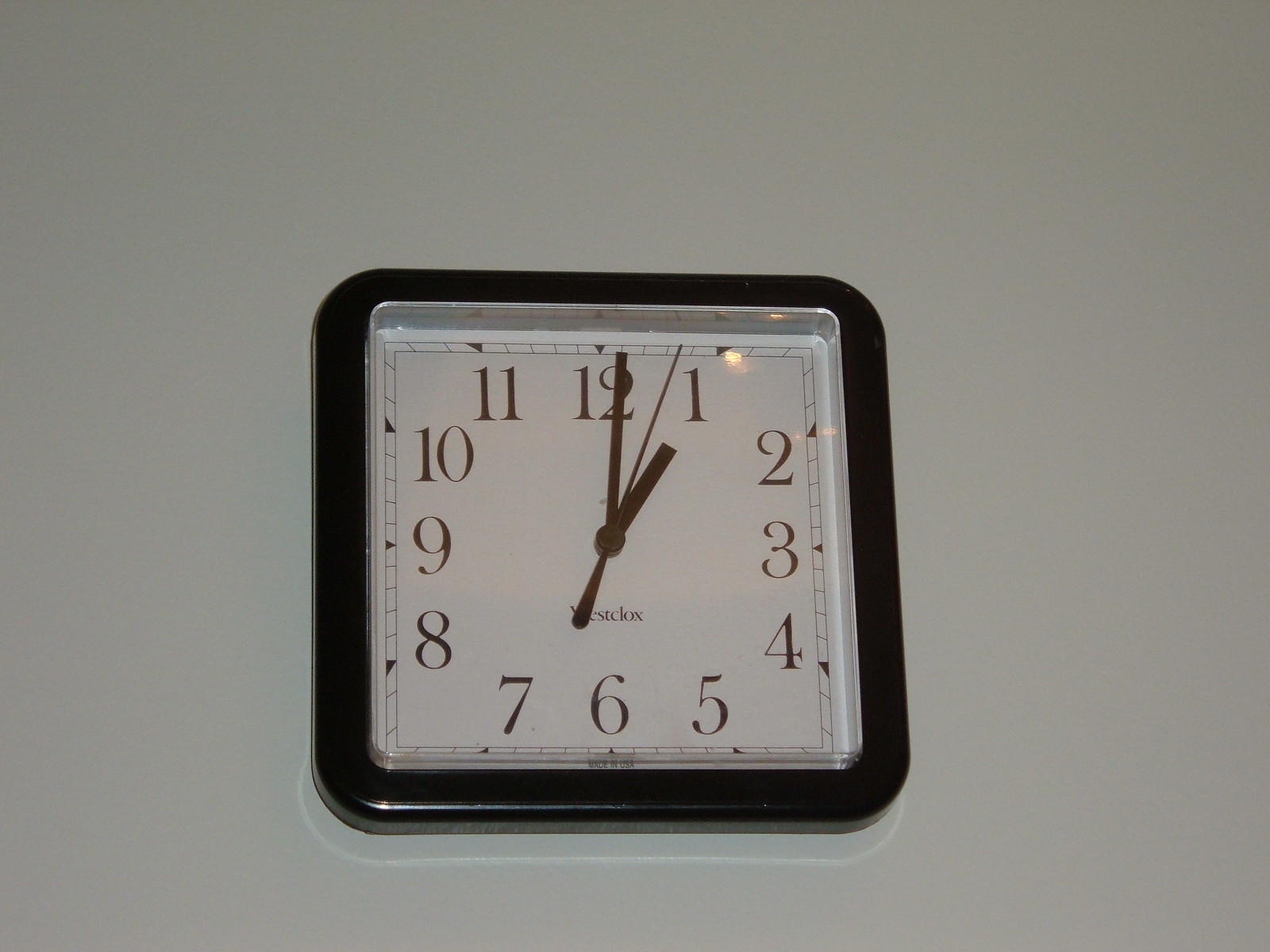A close-up image reveals a section of a white wall, prominently featuring a square-shaped clock mounted at the center. The clock itself has a distinguished black frame, while the dial inside is white, creating a distinct contrast. Clearly visible on the clock face are black numerals marking the hours 1 through 12. The clock hands, including the second hand, are also black, ensuring easy readability. Near the 6 o'clock position, partial branding is noticeable; some letters are obscured, but "E-S-T-C-L-O-X" is legible, suggesting that the complete brand name could be Westclox.